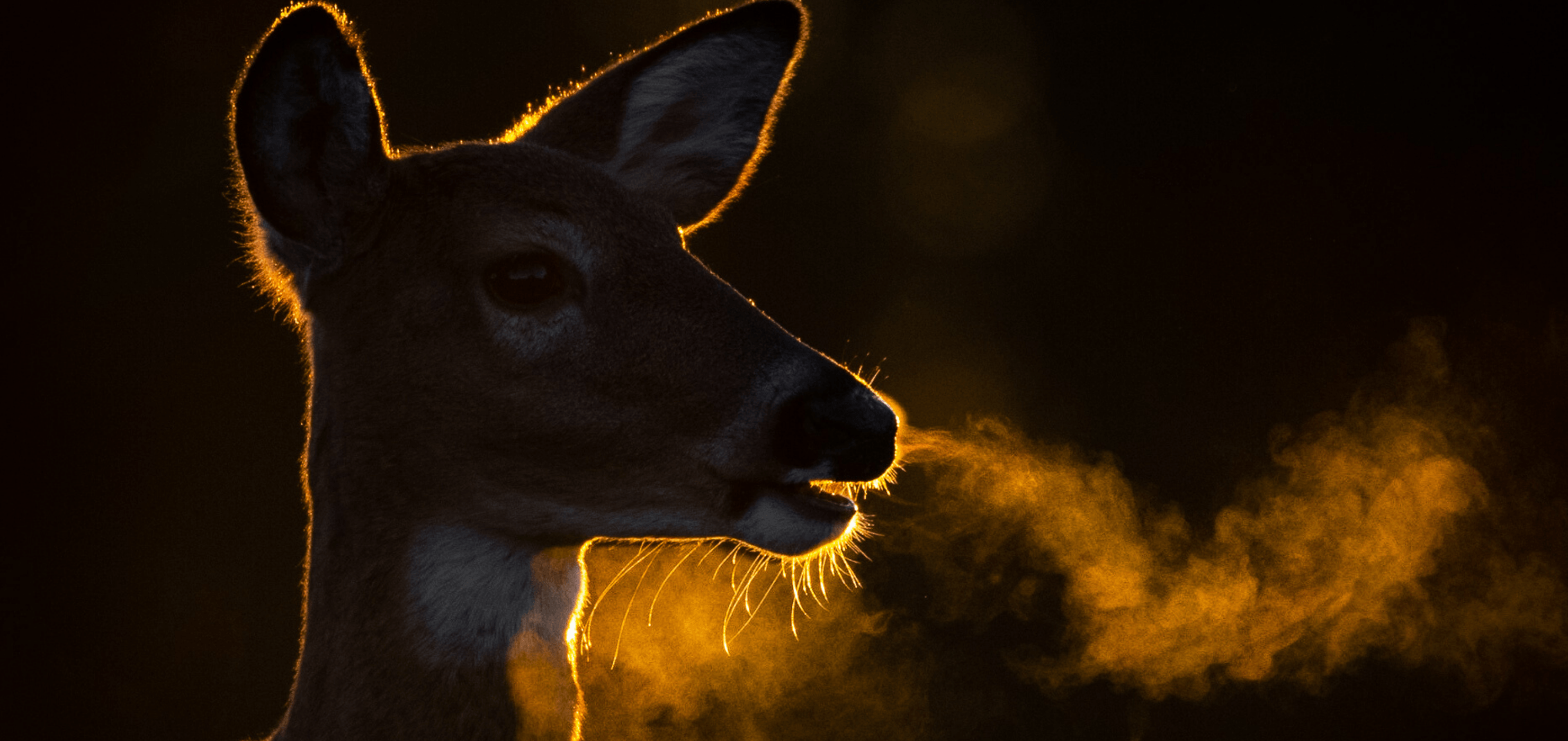The image depicts a deer, likely a fawn given its lack of antlers, set against a pitch-black background. Positioned in a side view, the deer’s face and part of its neck are visible, while the rest of its body is cropped out. The deer has large ears and distinctly black eyes surrounded by noticeable white patches. There are additional white markings around its nose, mouth, and under its chin. The snout is black, and the coat appears predominantly brown with some white areas. The deer’s mouth is slightly open, exhaling visible steam, which appears white and is highlighted on the right side and below the neck, suggesting it is a cold morning or night under moonlight. The deer’s breath is captured as a golden-hued mist due to the lighting, adding a mystical quality to the photograph.